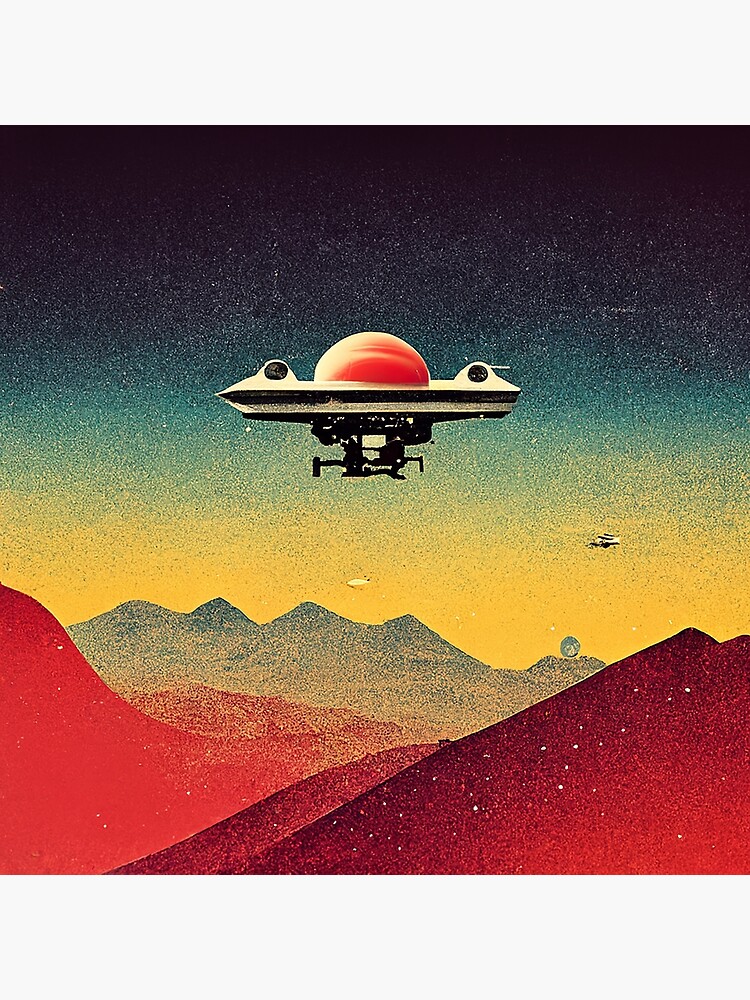This painting, likely done with watercolor or acrylic paint and employing a pointillism technique, depicts a highly futuristic scene. Dominating the center of the image is a floating, flying saucer-like observatory with a red dome on top, which has a beige reflective surface on its left side. Beneath the red dome are white, wing-like structures forming the main body of the spacecraft, and a mechanical black machinery forms its base. Surrounding this central saucer are additional, smaller spaceships scattered throughout the sky, with one notably positioned in the far background on the middle right. The sky itself transitions from a deep black at the top to a dark blue, eventually fading into yellow near the horizon. Below this celestial gradient lie layers of mountainous terrain—red mountains in the foreground contrasting against bluish-yellow and greenish mountains in the distance. The entire scene is rendered with a fine attention to detail, capturing the futuristic aesthetic amidst the tranquil yet otherworldly landscape.